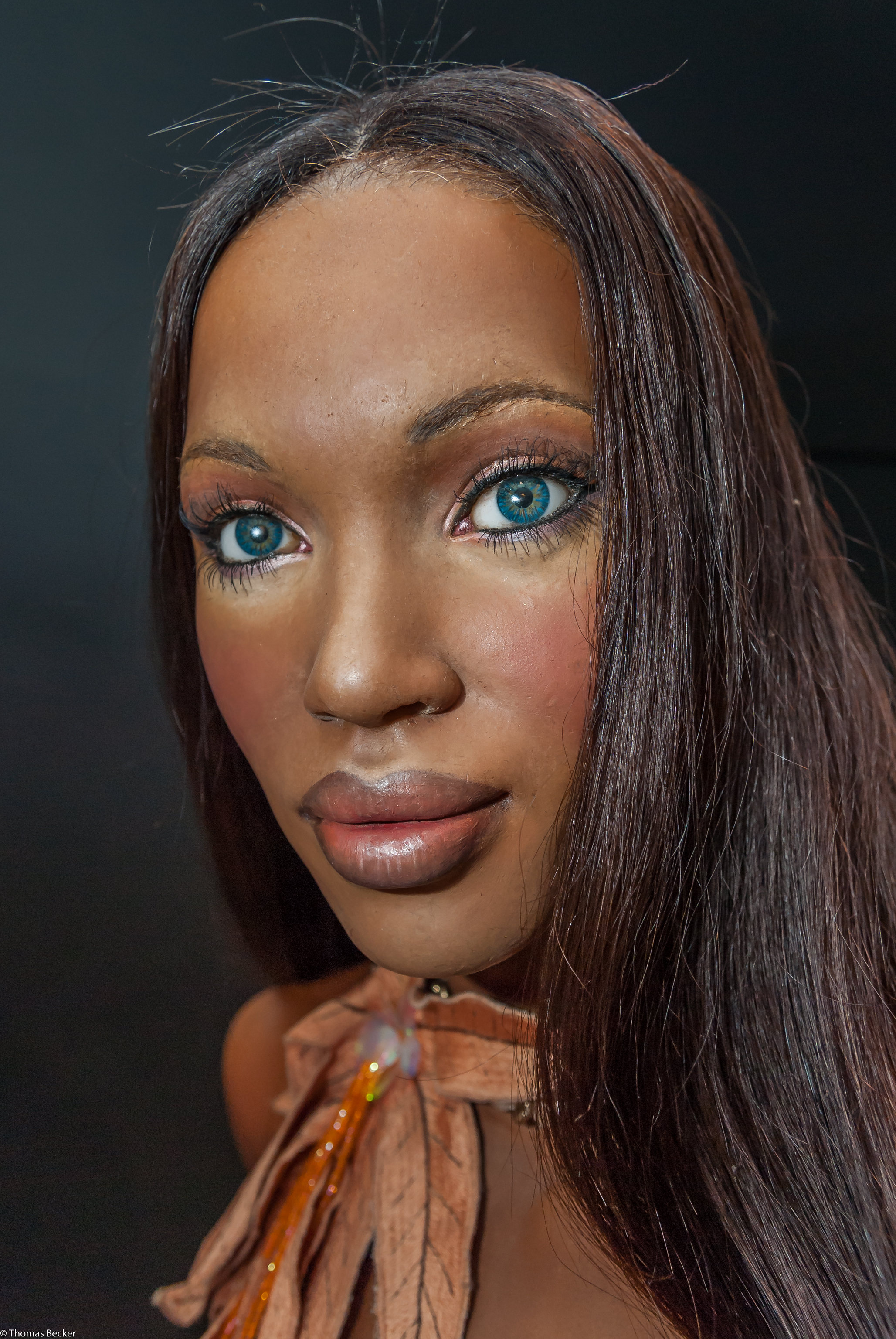The image features a close-up, vertical photograph of a striking black woman with long, slightly unkempt brown hair highlighted with reddish tones, parted down the middle with noticeable flyaways. She has captivating blue eyes, achieved through blue contacts, and wears heavy makeup, including vivid blush, prominent red lips with a darker lip liner, and intricate golden highlights outlining her eyebrows, cheeks, lip area, and the tip of her nose. Her eyes are accentuated with mascara and reddish eyeliner. The background is a dark, bluish-gray, providing a stark contrast to her detailed facial features. Under her chin, she wears or holds something resembling the leaves of a flower, in a tan or orange color, adding a distinct accessory to the image, although it is unclear if it is part of a scarf or her outfit.